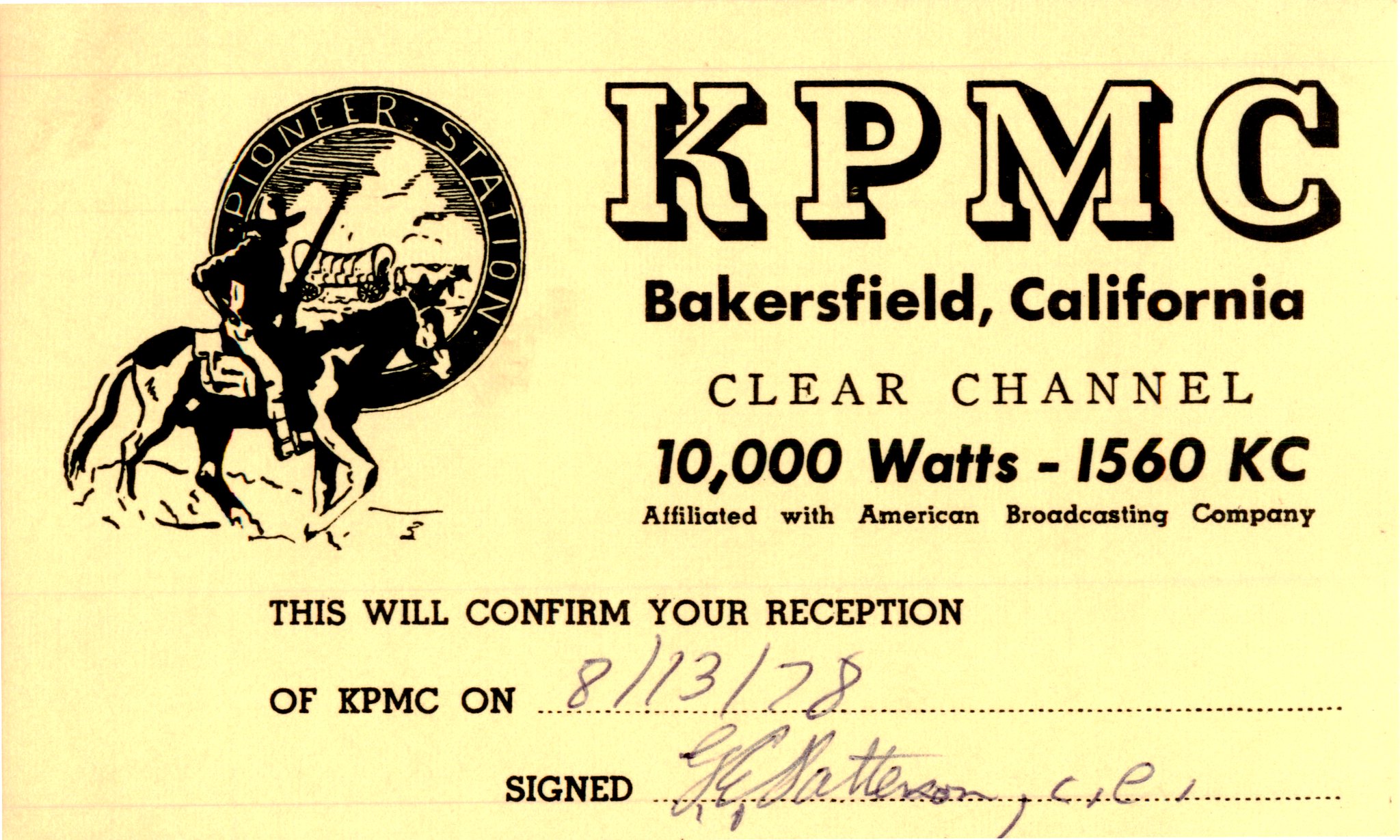The image features a vintage yellow card with prominent black text and a distinct emblem. In large bold letters at the top, it reads "KPMC". Below it, the card details "Bakersfield, California, Clear Channel, 10,000 watts, 1560 KC, affiliated with American Broadcasting Company". To the left, a circular emblem depicts an animated cowboy on horseback, accompanied by the words "Pioneer Station". Under this emblem, the text states, "This will confirm your reception of KPMC on August 13, 1978," followed by a handwritten signature on a line, possibly signed by someone with the last name "Matherson, CE".